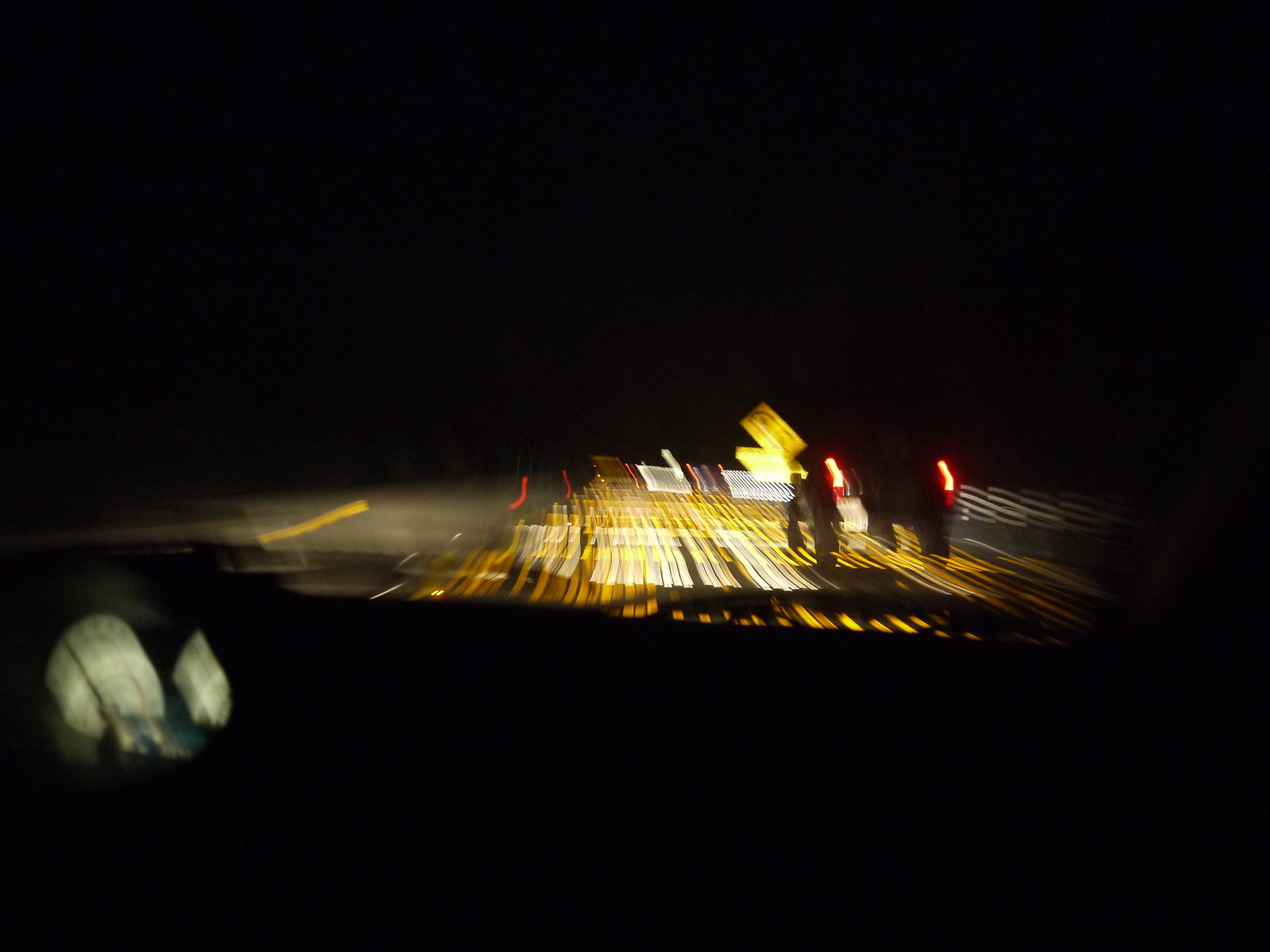The image depicts a night drive taken from inside a moving car while traveling down the interstate. The sky is pitch black, offering no ambient light except for the illuminated elements within and outside the vehicle. On the dashboard, you can see the lit-up gauges, particularly the speedometer on the right-hand side. The windshield wipers are faintly visible in the shadows at the center of the windshield.

In front of the car lies the roadway, where the motion blurs the visual elements, creating streaks of yellow from the lane markings and red from the taillights of another car in the right-hand lane. This adjacent car is only partially visible, primarily identifiable by its red taillights. There is also a yellow sign along the roadside, though it appears blurred and elongated due to the vehicle's movement. The headlights of nearby cars pierce through the darkness, adding to the sense of speed and motion captured in this dynamic, albeit blurry, night scene.